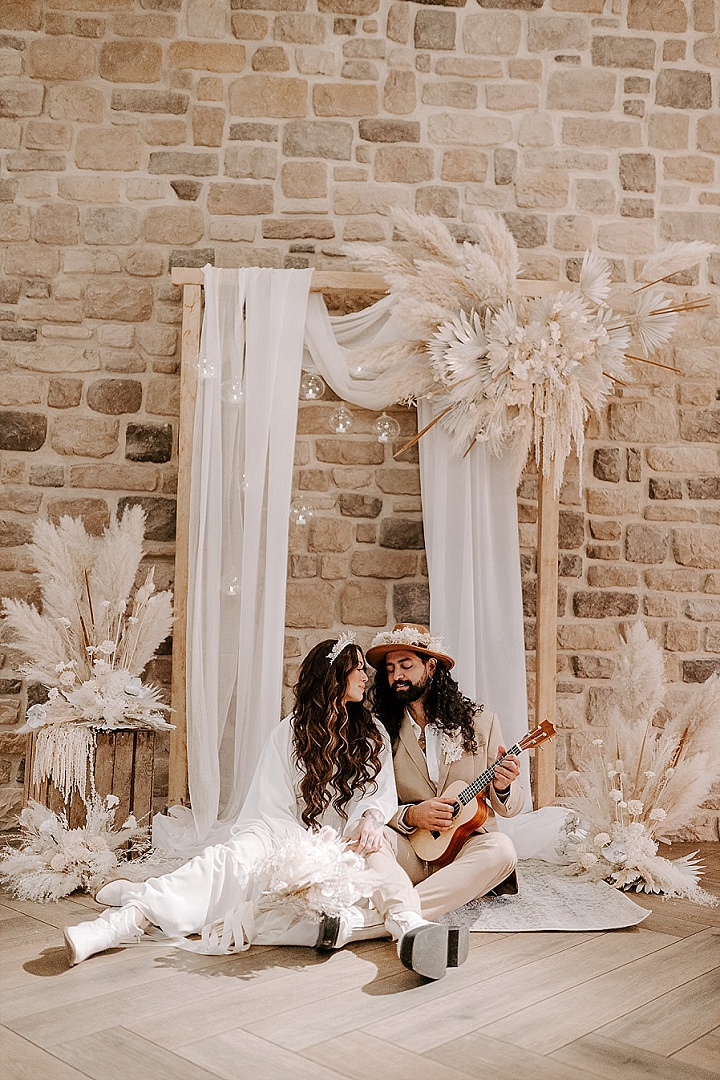In this color photograph, oriented in portrait, a couple dressed in wedding attire sits on a light-tiled floor, gazing affectionately at each other. The backdrop features a large beige stone wall. Behind them stands a simple wooden arch with a sheer, white lacy curtain draped over it. A unique floral arrangement, consisting of feathers and white paper flowers, decorates the top right corner of the arch, with smaller matching bundles on either side near the floor. Multiple glass discs hang overhead, adding an elegant touch.

The woman, seated on the left, is dressed in a flowing white gown and white boots, her legs crossed in front of her. She sports long, curly dark hair, adorned with a white pearl crown, and her serene gaze is directed at the man beside her. The man, sitting cross-legged, wears a tan suit and holds a wooden ukulele. He has long curly dark hair, a beard, and a straw hat adorned with white flowers. Both have their eyes lowered, contributing to the peaceful, intimate atmosphere of the image.